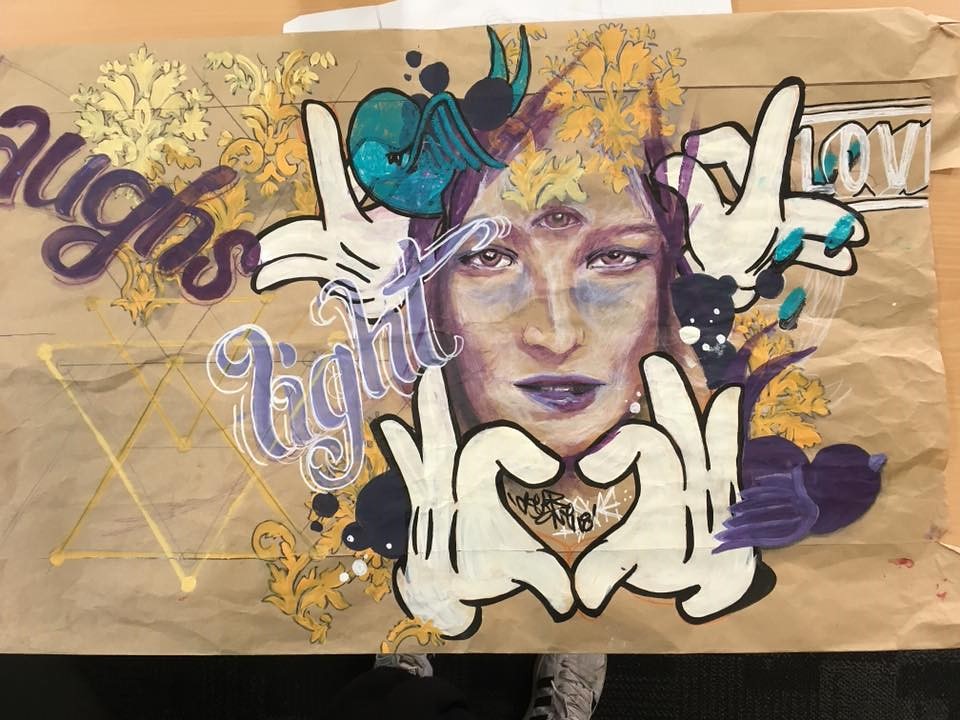This artwork, drawn on a textured brown paper, captures a surreal portrait of a woman. Central to the image is her face, adorned with three eyes – a third eye positioned on her forehead in addition to the standard pair. Her flowing hair and lips are vividly colored in shades of purple, adding a striking contrast to the composition. Beneath her face, two hands resembling the gloved hands of Mickey Mouse form a heart shape, each adorned with only three fingers and a thumb. These distinctive white gloves are mirrored on either side of her forehead, with fingers pointing upwards. The word "light," sketched in blue, is placed to the left of her face, suggesting a thematic element. Surrounding the woman are intricately drawn gold leaves, enhancing the mystical aura of the drawing. On the right side, a delicate purple bird perches, complementing the color palette and adding a touch of whimsy to the surreal scene.